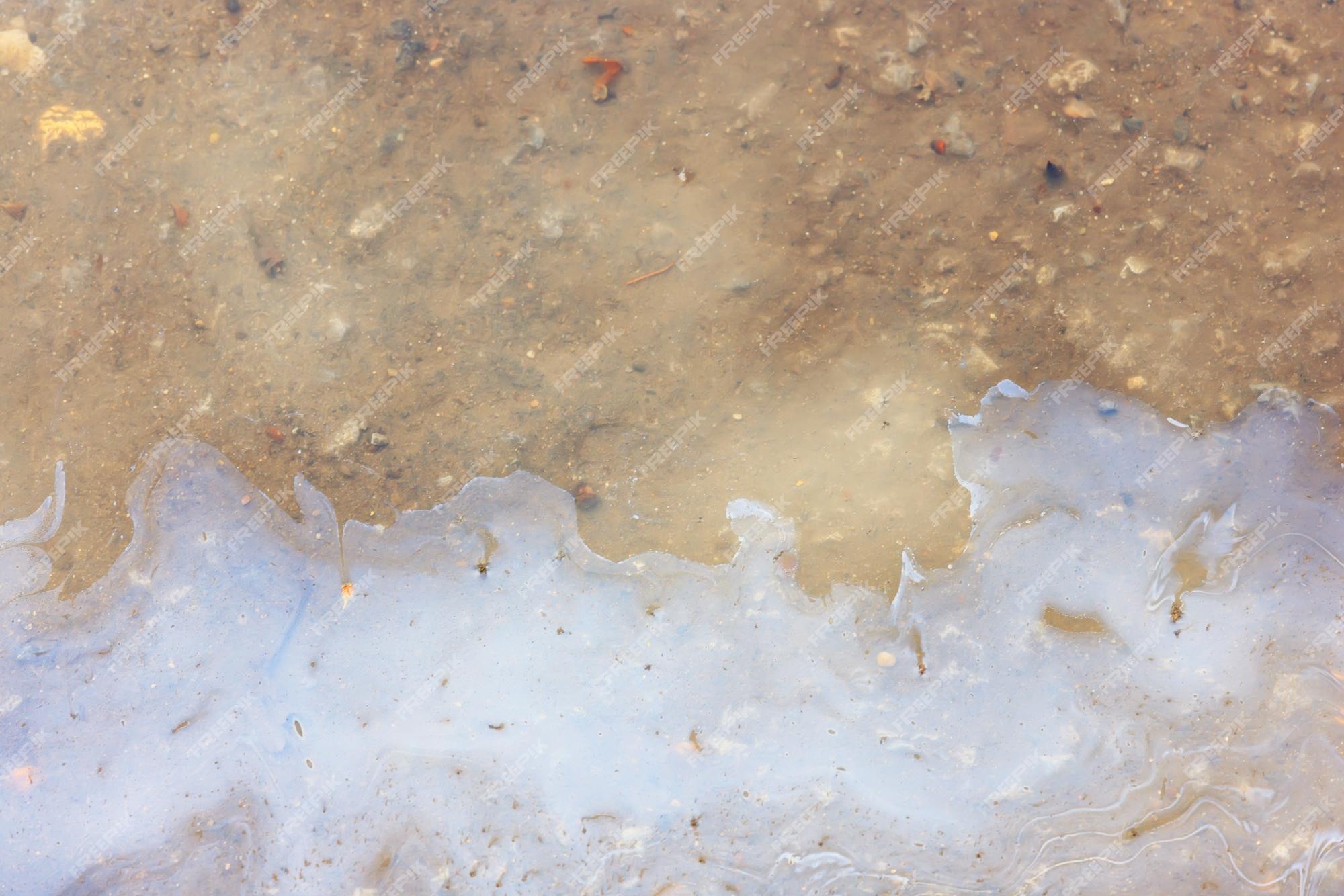The image features a close-up view of a reddish-brown dirt surface mixed with small rocks and pebbles. Along the bottom portion of the image, there's a spill of creamy-colored liquid, resembling a mixture of dish soap and water or milk, forming a boundary with the dry dirt above. This liquid spill creates an impression of shallow water over the dirt. Around the center of the image, a hazy effect is present, possibly due to the color of the dirt or an artifact in the photograph. The image also includes an overlay of copyright text, running diagonally in several rows from bottom to top, repetitively reading "Freepik."